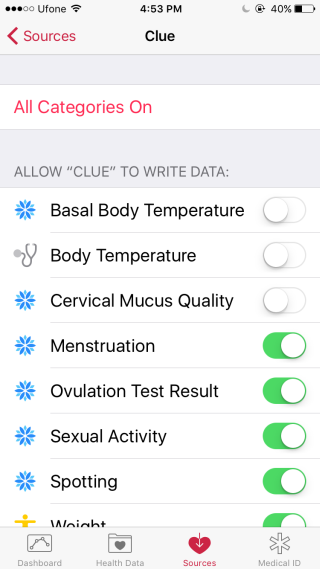This image appears to be a screenshot of a health tracking application on a smartphone.

At the top of the screen, the status bar is visible, showing several icons and indicators. From left to right, there are three solid and three checked circles next to the Uphone icon, indicating some form of status or progress. To the right of that, there's the Wi-Fi symbol, followed by the time displayed as 4:53 PM in the center. Further to the right, there are icons indicating the phone is in Do Not Disturb mode (moon icon), the screen is locked (lock icon), and the battery level is at 40%.

Below the status bar, there is a red back arrow and the app's interface. The header is colored red and labeled "Sources". In the center, it says "Clue".

The app's main interface appears on a white background with various sections. Below the red header in red text, it says "All Categories On," followed by a gray field instructing "Allow 'Clue' to write data."

The interface features several health tracking options, each with an associated icon to the left. Most of these icons are snowflakes, except for a stethoscope for body temperature and a yellow person icon at the bottom. There are sliders to the right of each option, indicating whether they are toggled on or off. The first three sliders are off, while the next five are on. The categories listed are:

1. Basal Body Temperature (off)
2. Body Temperature (off)
3. Cervical Mucus Quality (off)
4. Menstruation (on)
5. Ovulation Test Results (on)
6. Sexual Activity (on)
7. Spotting (on)
8. Weight (on, but cut off)

At the bottom of the screen, there are four navigation icons. From left to right:

1. A graph labeled "Dashboard."
2. A heart on a folder labeled "Health Data."
3. A red heart labeled "Sources," which is currently highlighted.
4. A medical ID with a six-pointed star symbol.

This detailed layout suggests the app is designed to track various aspects of women’s health, providing a comprehensive overview via a user-friendly interface.